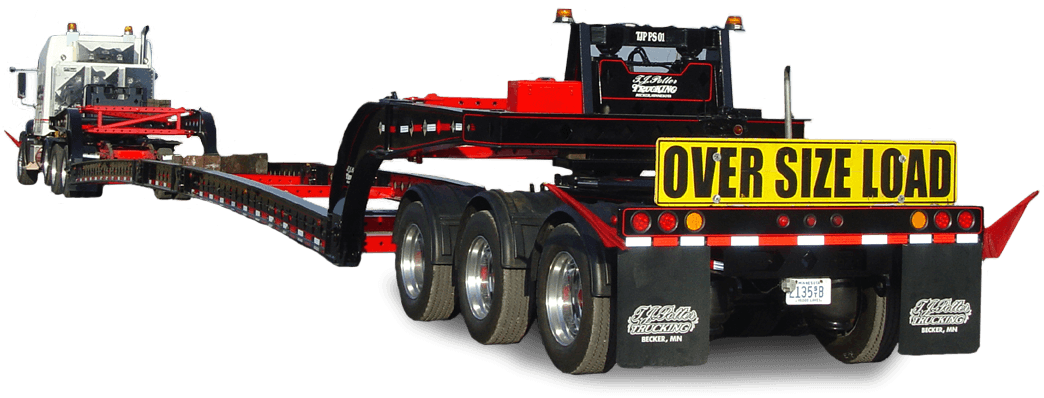The image features a semi-truck with a completely white, photoshopped background, making it appear isolated from any setting. The truck, positioned towards the left side and facing away from the camera as if driving away, boasts a bright white cab. On top of the cab are a couple of orange lights. The truck hauls an extremely long trailer, predominantly painted in red and black, with three sets of tires at the rear. Notably, the trailer has a large yellow sign with black lettering that reads "Oversize Load" above the red and orange tail lights. The bed of the trailer seems to be mostly empty, with perhaps a few logs positioned near the front. The front of the truck is visible in the distance, anchored at the top left corner of the image, emphasizing the expansive length of the vehicle. The trailer’s robust, curved metallic frame is prominently on display, underlining its capacity for heavy-duty loads. The color palette of the scene includes yellows, oranges, reds, whites, and variations of black, contributing to the vivid yet industrial aesthetic of the photograph.